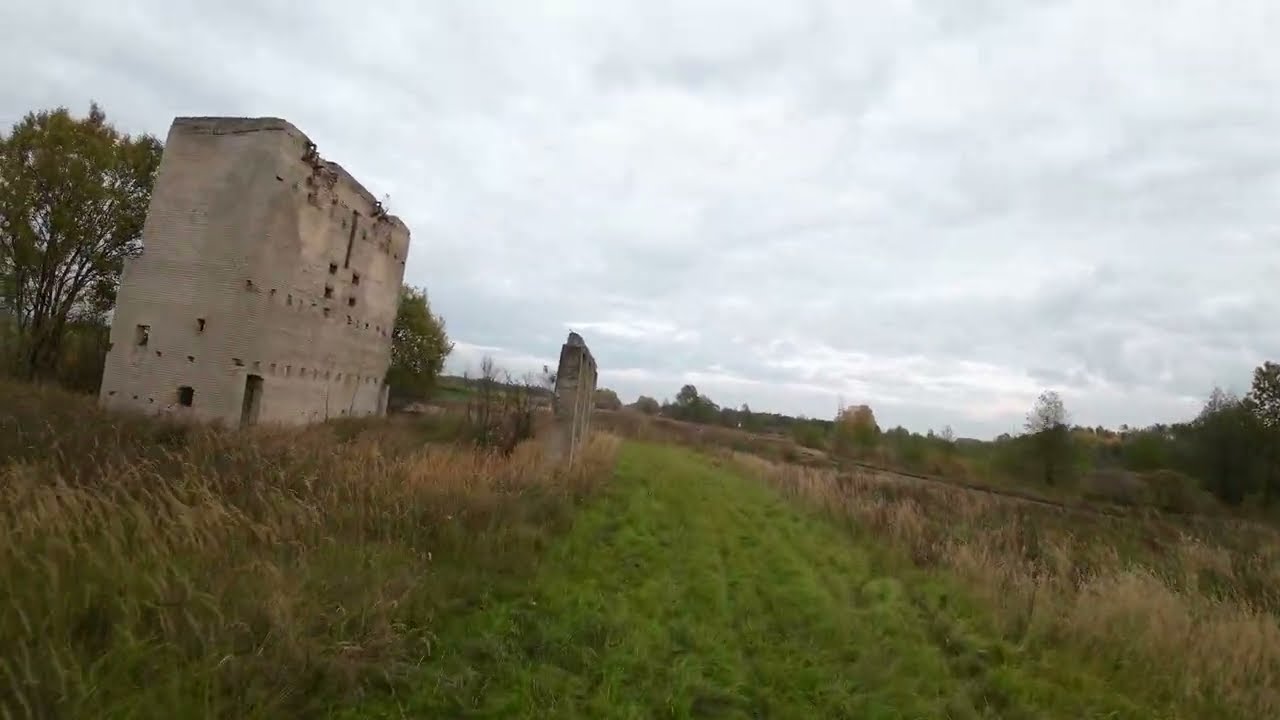The photograph captures an outdoor scene featuring a large, derelict building set within a predominantly green, unmowed field. A grassy path, slightly mowed in comparison to the surrounding taller and browner grass on either side, extends from the foreground and curves gently to the left around the structure. The building, appearing to be made of weathered concrete or stone, stands a couple of stories tall with door and window openings carved into its facade, indicating significant wear and age, possibly hinting at a past military use. In front and to the right of this structure, a series of disconnected concrete pillars suggest remnants of a once larger complex that has since deteriorated. To the right of the grassy path, a street or road is visible, bordered by a dense cluster of trees in the distance. The sky overhead is overcast and gray, with heavy clouds hinting at imminent rain, contributing to the overall gloomy atmosphere of the scene.